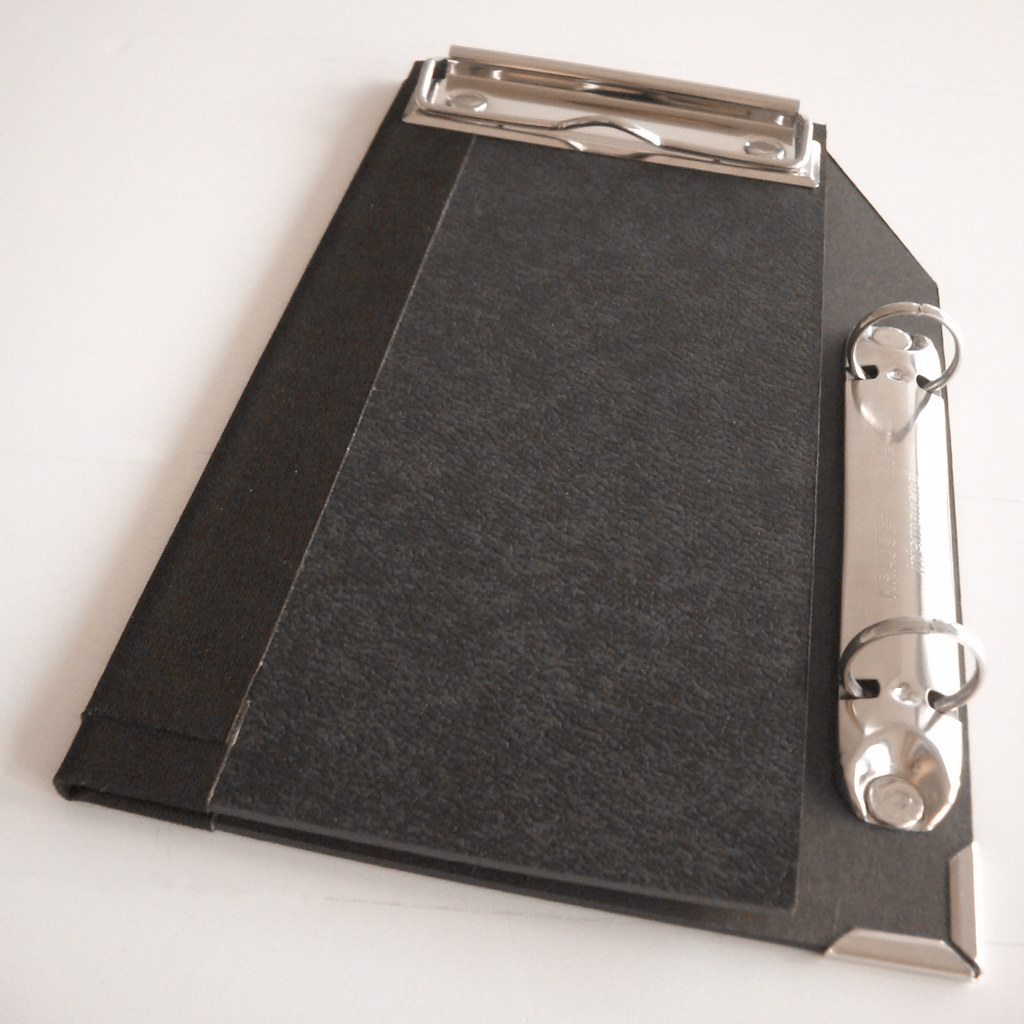The image depicts a distinctive clipboard, crafted from black pressboard material with a textured finish. This clipboard is characterized by a heavy black binding that secures its two folds, giving it a sturdy construction. Dominating the top section, there is a spring-loaded metal clasp, featuring a slight bend in the middle—designed for easy finger access—to securely hold papers. On the right side of the clipboard, a metal plate is riveted to the board, integrating two ring binders that can accommodate two-ringed hole-punched paper. These ring binders open at the center, allowing for easy insertion and removal of documents. Additionally, the clipboard includes a metal bracket at the bottom right-hand corner, serving as a protective device against accidental impacts. The entire assembly rests on a white table or countertop, presenting a sleek, functional design that merges both clipboard and binder functionalities.